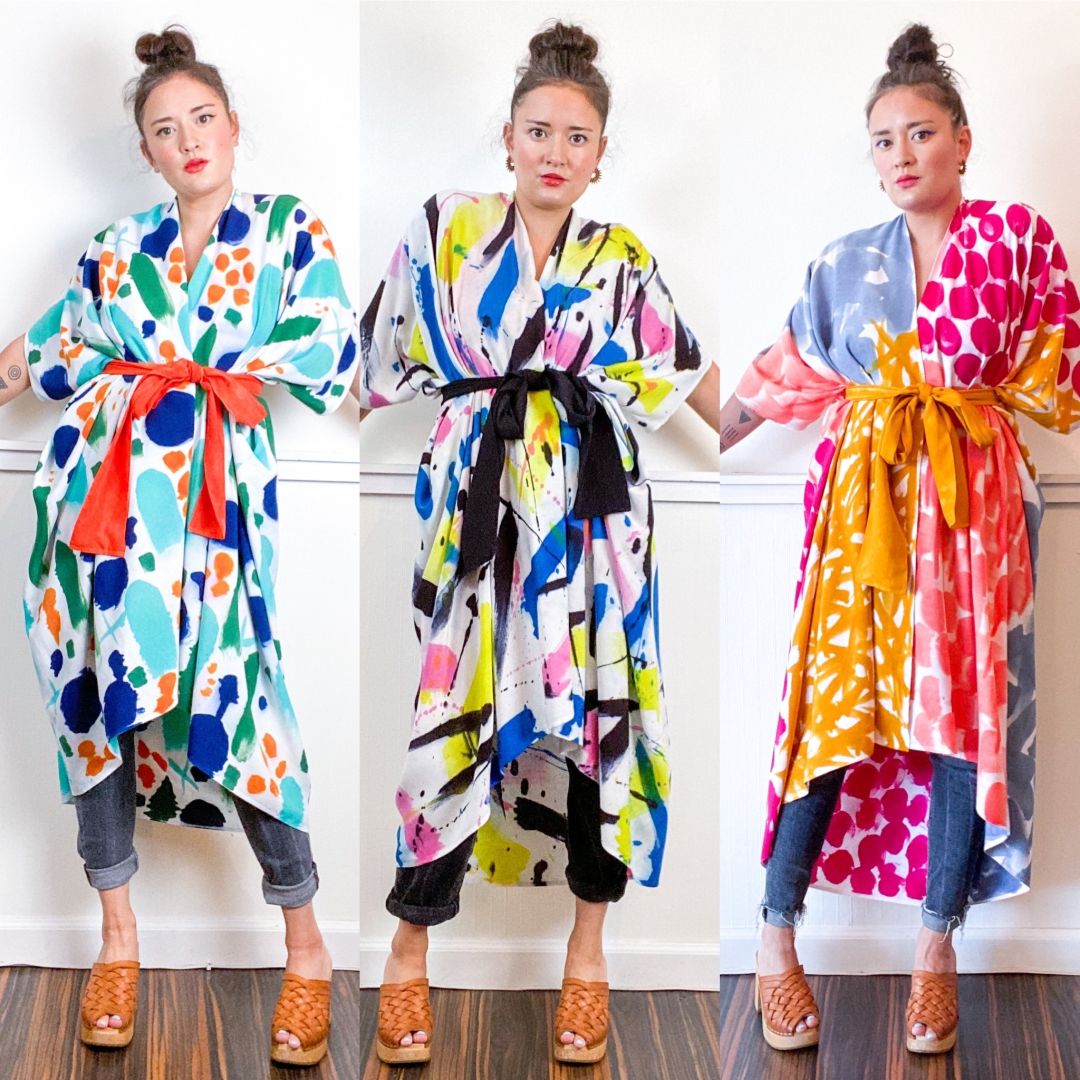This image showcases a woman modeling three vibrant kimonos, standing against a white wall on a dark wooden floor. Her hair is styled in a bun and she wears the same brown, open-toed platform shoes in each photo. The kimonos, which exhibit a watercolor-like abstract pattern, vary in color and detail:

1. In the first kimono, she sports rolled-up blue jeans. The white robe is adorned with diverse patterns, including orange and blue dots, green strokes, and turquoise ovals, and is cinched with an orange sash.

2. In the second kimono, she wears rolled-up black pants. This white robe features paintbrush-like streaks in blue, pink, yellow, and black, and is tied with a black belt.

3. In the third kimono, she wears longer blue jeans. The robe showcases a mix of pink, orange, peach, and blue dots and lines, and is fastened with a gold sash.

Across all three images, the model maintains a neutral expression, highlighting the detailed and colorful patterns of each kimono, which resemble abstract paintings.